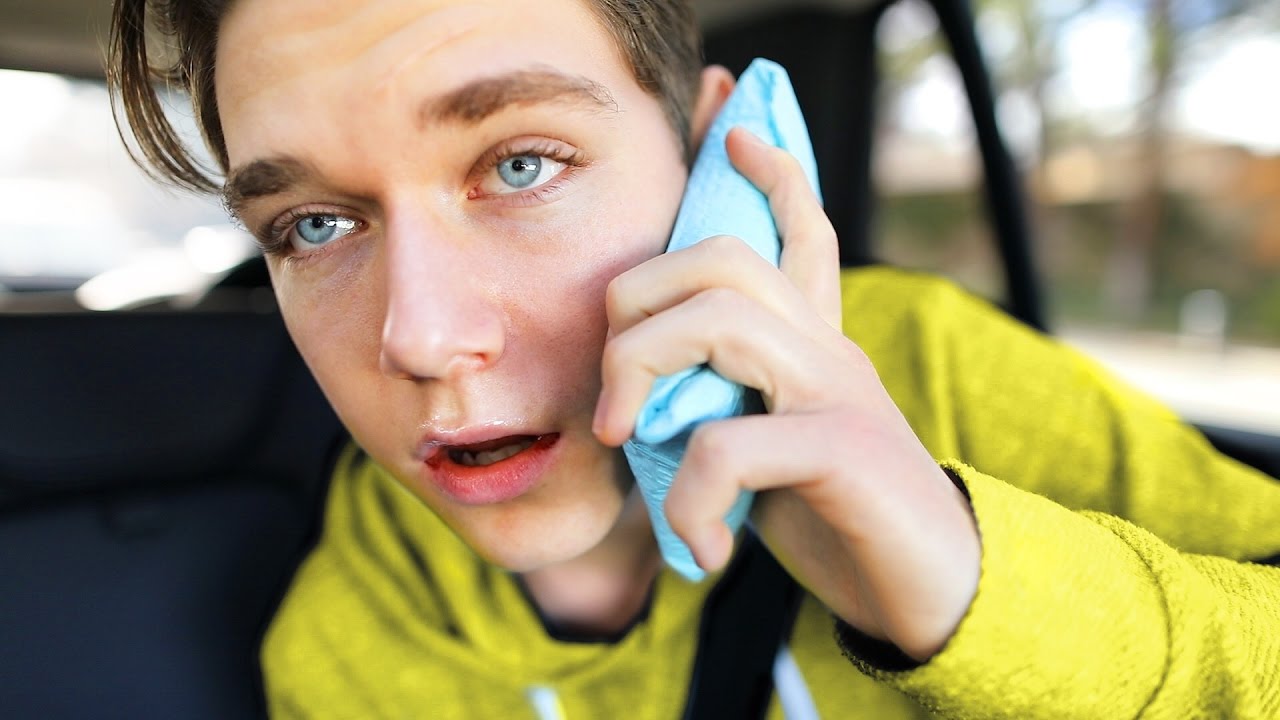This close-up, professionally-shot photograph, in color and horizontal format, captures a young man, likely a teenager, seated in what appears to be the backseat of a car, with a blurred background that hints at trees and buildings without providing specific details. He's wearing a yellow (or lime green) hoodie with white hood ties, and a seatbelt is visible. The young man holds a blue object—possibly a phone or an unusually shaped phone case—up to his left ear. His mouth is slightly parted, and his expression is somewhere between curious and glazed, as he gazes off to the left of the photograph, just over the photographer's ear. His eyes carry a distant, almost dreamy look, adding an ambiguous emotional layer to the portrait. The interior of the car seems dark blue, contrasting with the young man's white skin and bright hoodie.